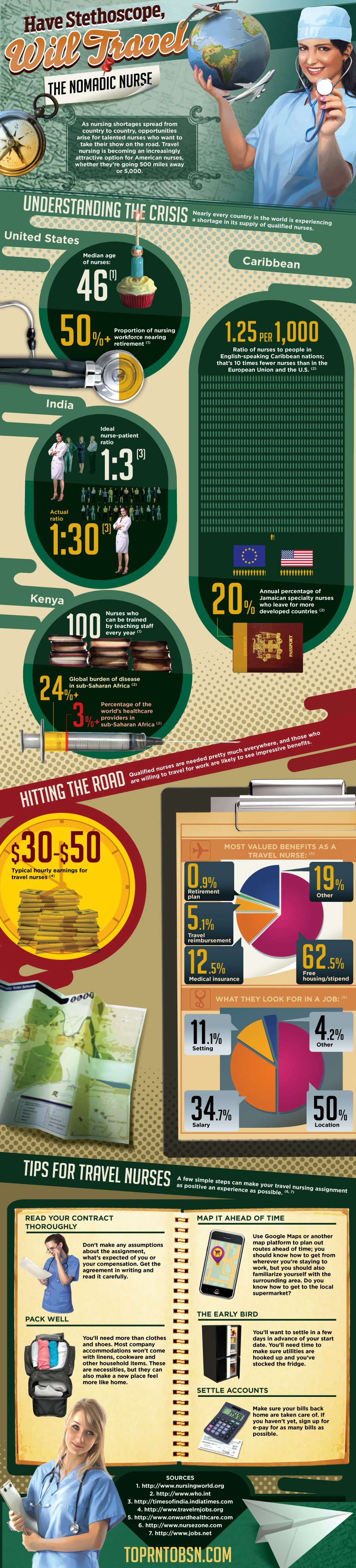### Caption:

**Top RN: Travel Nursing Opportunities and Benefits Revealed**

An in-depth advertisement highlighting the lucrative and adventurous career of travel nursing. At the top, the slogan reads: *"Have Stethoscope, Will Travel. It's the Nomadic Nurse."* The main image features a confident nurse in blue scrubs with blonde hair, holding a notepad and a stethoscope draped around her neck. She stands ready to embark on her next assignment, exemplifying the essence of a dedicated travel nurse.

The ad provides several key pieces of advice for aspiring travel nurses:
- **Read your contract thoroughly.**
- **Pack well.**
- **Map it ahead of time.**

These tips are emphasized with phrases like *"The early birds settle accounts."*

Further informational graphics include:
- **Typical Hourly Earnings for Travel Nurses**: Displayed in a burgundy circle, indicating $30 to $50 per hour.
- **Sources of Information**: Websites such as nursingworld.org are credited.

The detailed pie charts illustrate:
- **Travel Nursing Benefits Breakdown**: 
  - Free Housing: 62.5%
  - Medical Insurance: 12.5%
  - Travel Reimbursement: 5.1%
  - Retirement Plan: 0.9%
  - Other: 19%

- **Key Job Considerations**:
  - Location: 50%
  - Salary: 34.7%
  - Setting: 11.1%
  - Other: 4.2%

Global nurse statistics are highlighted:
- **Ratio of Nurses to People**: 1.25 per 1,000 in English-speaking Caribbean nations—ten times fewer than in the EU and the US.
- **Annual Percentage of Jamaican Specialty Nurses Leaving for More Developed Countries**: 20%.
- **Median Age of Nurses**: 46 years.
- **Proportion of Nursing Workforce Approaching Retirement**: 50%.

A noteworthy circle graph mentions the ideal nurse-to-patient ratio, which is 1:3, with emphasis on the actual ratio being somewhat different.

The ad emphasizes the global demand and shortage of nurses, pointing to vast opportunities for those willing to travel. It portrays an adventurous image of a nurse with a stethoscope in her ears, holding a world globe with airplanes circling, symbolizing the nomadic lifestyle and myriad opportunities available.

Lastly, this well-rounded and comprehensive ad aims at attracting skilled nurses to take their careers on the road, promising high pay, extensive benefits, and significant personal growth.